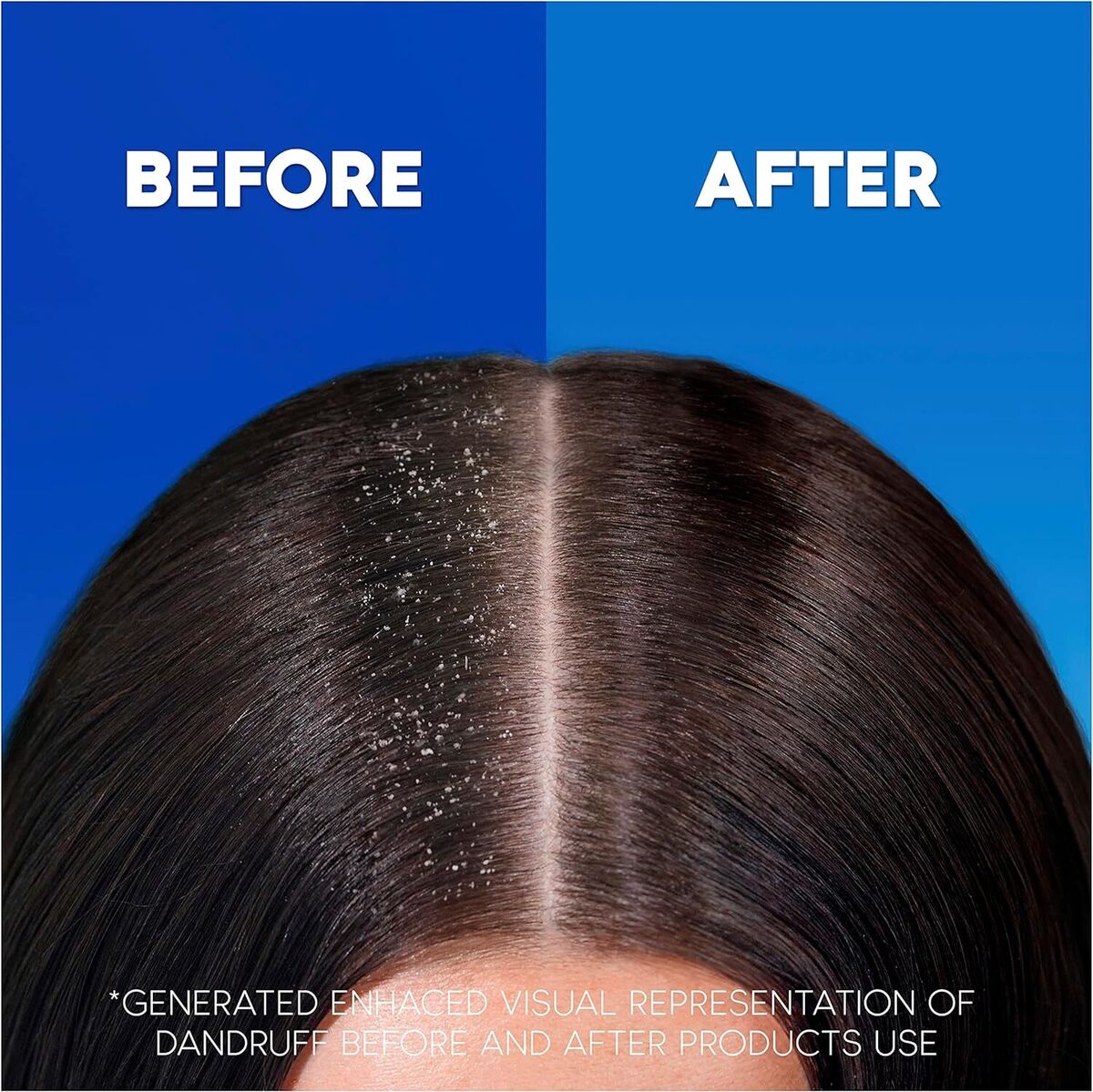This image is a detailed, split-screen, color photograph of the top of a woman's head, designed to showcase a before and after comparison of dandruff treatment. The woman has dark, black, straight hair, parted precisely down the middle, revealing the top section of her forehead at the bottom center. On the left side of the split image, set against a dark blue background, her black hair is covered with numerous white flakes of dandruff and the word "before" is displayed in large white text at the top corner. Contrasting this, the right side features a light blue background with visibly smooth, dandruff-free hair and the word "after" is similarly displayed. At the bottom, a disclaimer in smaller white text with an asterisk reads "generated enhanced visual representation of dandruff before and after product's use." Despite not specifying the product used, the image effectively illustrates the reduction in dandruff.